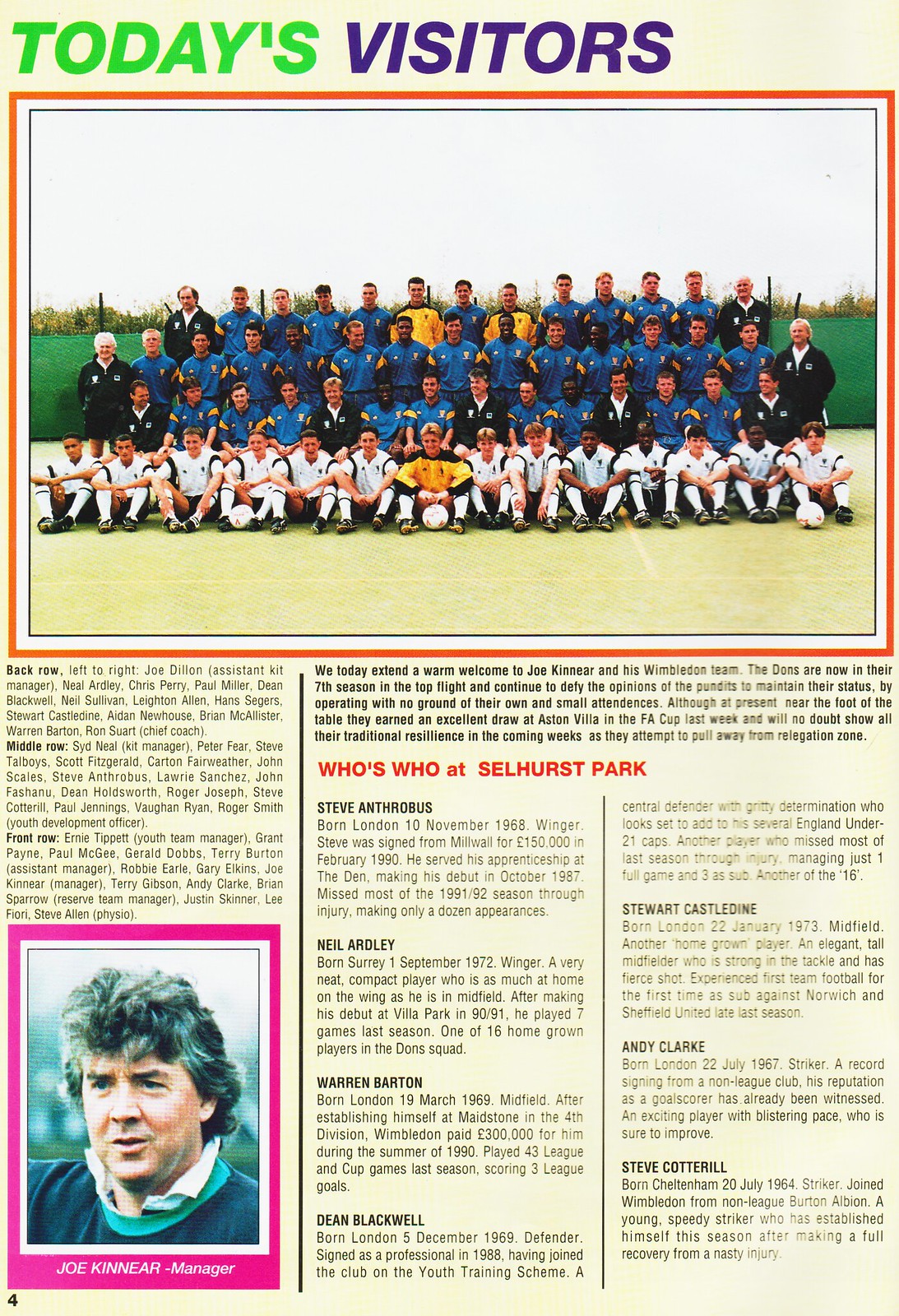The image depicts an old newspaper or magazine article featuring a soccer team. Centrally placed is a team photo arranged in four rows; the first row showcases players in white jerseys sitting on the ground, including one in a yellow and black jersey. The second row, seated as well, mainly features players in blue and yellow jerseys with a few in black. The back two rows consist of standing players predominantly donning blue and yellow jerseys, with some in black and a few in yellow. Standing on the corners and sides are several coaches.

Above the image, bold text reads "Today's Visitors," with "Today's" in green and "Visitors" in blue. Below the image lies a dense block of text in three columns on a faded white background, printed in black font. Each column contains descriptive paragraphs about different players, including Anil Eldarai, Warren Barton, Dean Blackwell, among others. There are mentions of notable figures such as Steve Anthrobus, Neil Ardley, Warren Barton, Dean Blackwell, Stuart Castledine, Andy Clark, and Steve Cotterell. Additionally, the photo includes a caption naming everyone present, and a smaller photo of the manager, Joe Kinnear, is located in the bottom left-hand corner. The context hints at this being part of a soccer magazine providing information about the team and its players, potentially under a heading like "Who's Who at Selhurst Park."